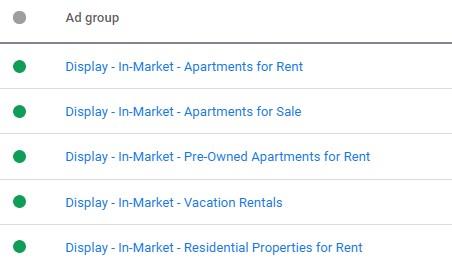The image features a simple, structured layout on a white background. At the top, there is a small gray circle, and to its right, bold black text reads "ad group." A horizontal black line separates this top section from the rest of the content.

Below the dividing line, five green circles of the same size as the initial gray one are aligned vertically. Each green circle is accompanied by blue, hyperlink-styled text to its right, listing various display options:

1. **display-in-market-apartments-for-rent**
2. **display-in-market-apartments-for-sale**
3. **display-in-market-pre-owned-apartments-for-rent**
4. **display-in-market-vacation-rentals**
5. **display-in-market-residential-properties-for-rent**

A thin gray line separates each option, enhancing the neat and organized appearance. Overall, the image appears to be a compact and cleanly-designed interface, possibly for a digital marketing or advertising platform.